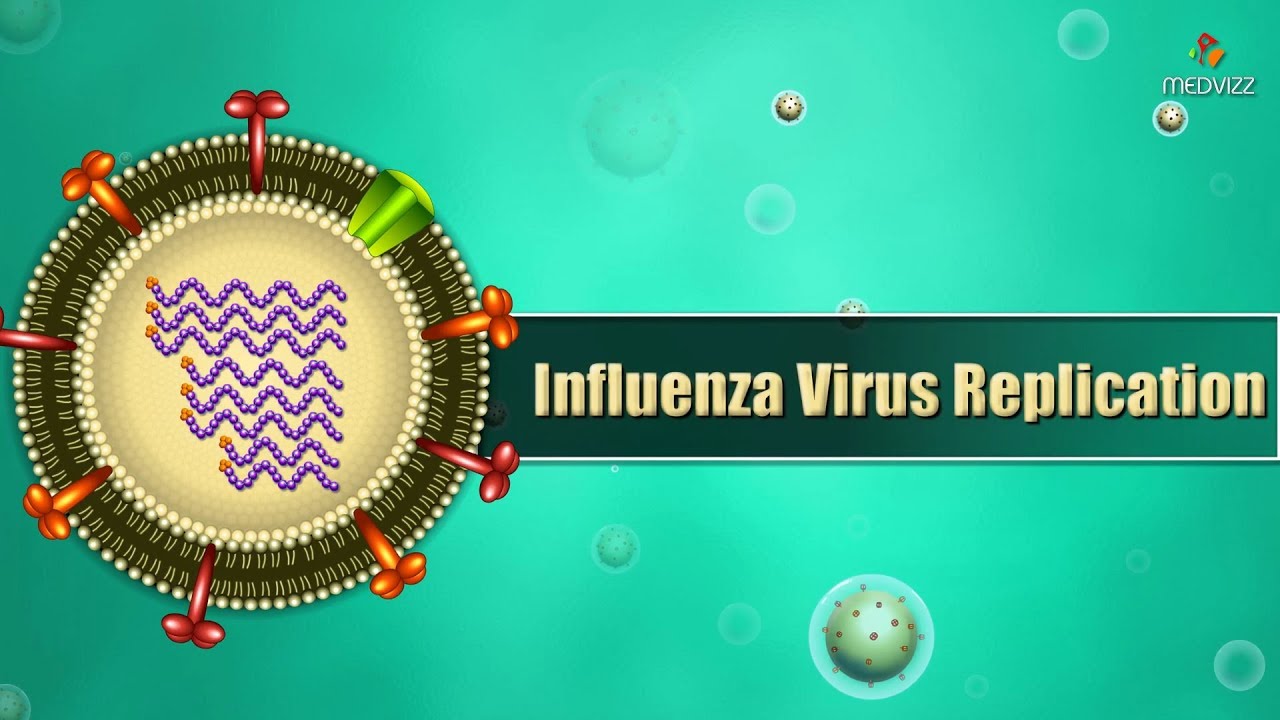The digitally illustrated image, reminiscent of a medical diagram or a PowerPoint slide, features a detailed representation of the Influenza Virus Replication process against a turquoise, or green, background. Dominating the center, the title "Influenza Virus Replication" is prominently displayed in yellow writing. At the top right corner, the label "MEDVIZZ" is inscribed in white writing, possibly indicating the software or company behind the illustration. Within the image, a large circular cell is depicted with dark brown borders and gold writing inside. This cell is adorned with red and orange prongs sticking out, and it contains intricate orange and purple squiggly lines and structures resembling viral RNA. Surrounding the main cell, several smaller green spherical cells with spiked protrusions float against the background, contributing to the scientific and educational aesthetic of the image.